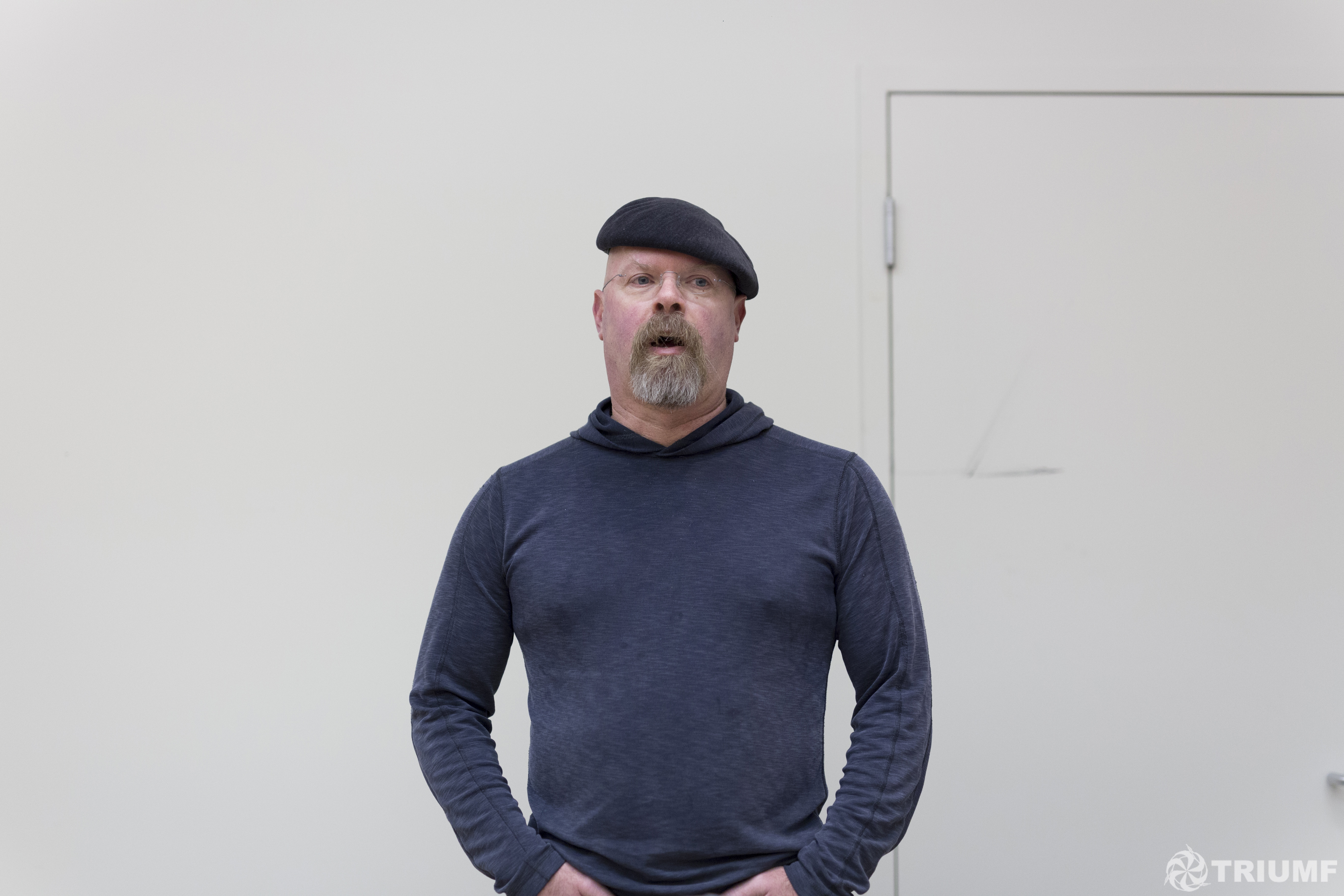The photo features a white male, seemingly in his 40s or early 50s, with a bulky frame and a thick head. He wears a navy blue long-sleeved hoodie made of a thin, T-shirt-like material, with the hood down around his neck. On his head is a matching navy blue beret, under which he appears to be bald or with his hair completely tucked in. He sports thin eyeglasses and a very bushy goatee with a brownish mustache and gray chin. The man, positioned centrally in the photo, has his hands possibly in the pockets of his jeans, and is looking slightly off to the right with his mouth open, as if speaking. The background is a plain white wall with a large white door to the right. The setting appears to be indoors, possibly in a living room, with the watermark "Triumf" and a circular vortex logo in white visible at the bottom right of the image.